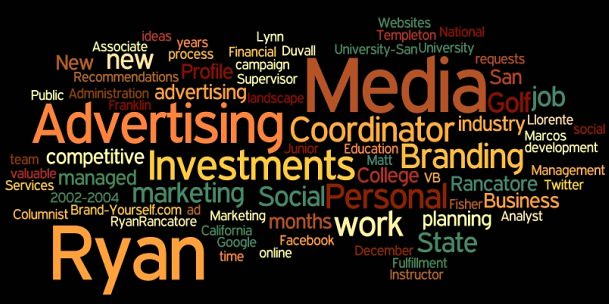The image features a vibrant, multicolored word cloud set against a black background. Various words and phrases, primarily related to advertising, marketing, and business, are scattered across the image in different fonts and colors, including orange, green, yellow, red, and blue. Notable words include "advertising" prominently in orange, "marketing" and "social" in green, "media," "coordinator," "branding," "planning," and "business." Names such as "Ryan," "Lynn," and "Deval" are also present alongside terms like "work," "state," "Google," "Facebook," "industry," and "associate." Institutions like "Templeton University" and "San University" are mentioned, portraying an intricate collage of terms typically associated with careers, digital presence, and professional development.